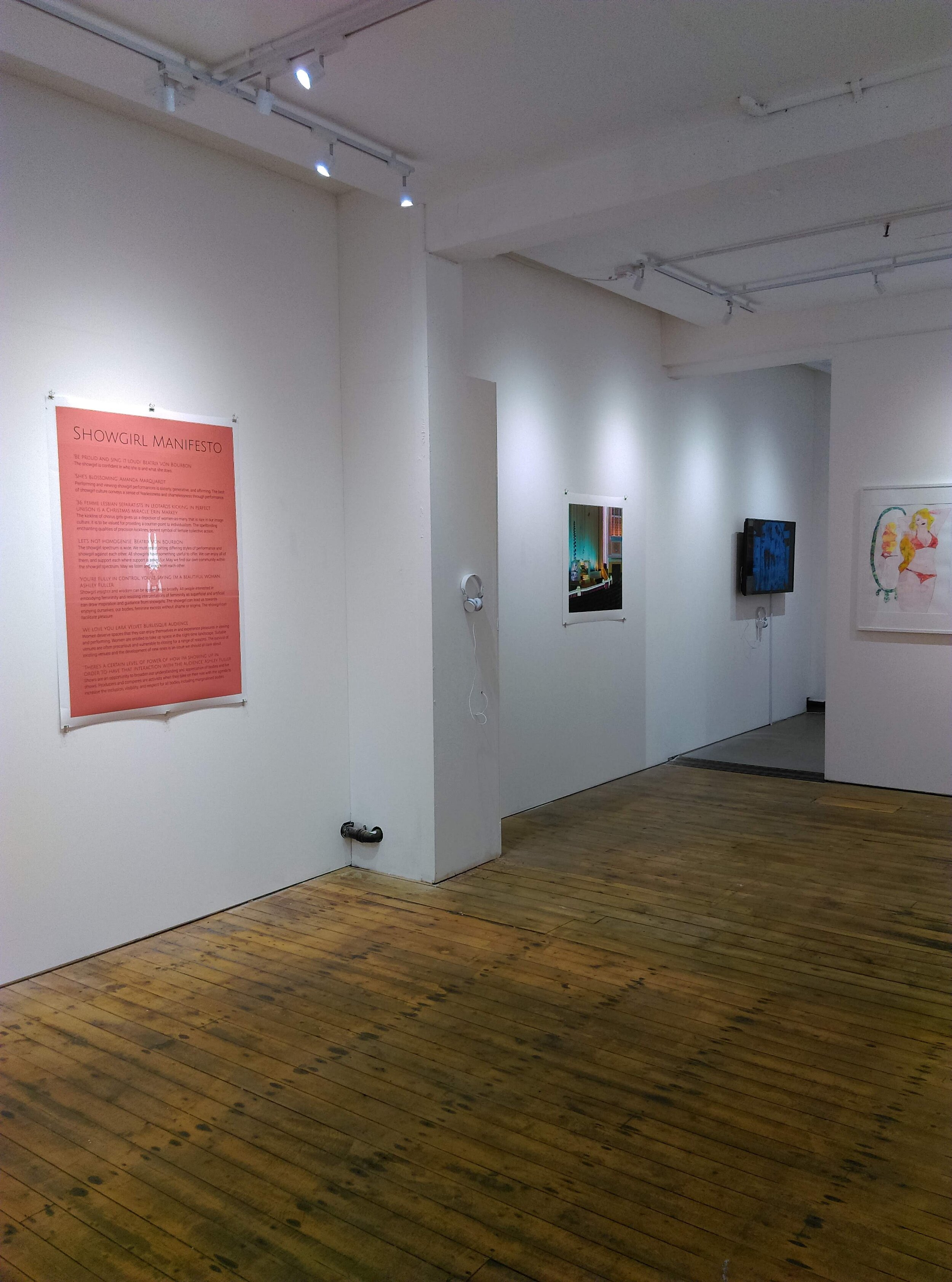The photograph captures a modern, minimalistic art gallery characterized by stark white walls and a wooden floor that showcases a prominent grain pattern. The lighting consists of track lights, precisely illuminating the artworks displayed on the walls. At the forefront is a poster titled "Showgirl Manifesto," printed in red text on a light red background and encased in glass or plexiglass, which possibly reflects an image or superimposes a woman doing a handstand over the text, though the manifesto's details are unreadable.

A dividing pillar or wall with a doorway separates two rooms, featuring an image of a blonde woman in a red bikini standing in front of an oval mirror. The woman faces away from the mirror, showing only the back of her head in the reflection. 

Other visible artworks include a distant photograph of what might be a city scene and another piece featuring shades of blue against a black background, which could resemble a flower. The gallery, likely a rented space for showcasing and selling art, is notably empty and arranged to minimize visual distractions, allowing each piece to stand out individually. A far-back room contains an LCD screen, connected to the wall, though its display remains indiscernible.